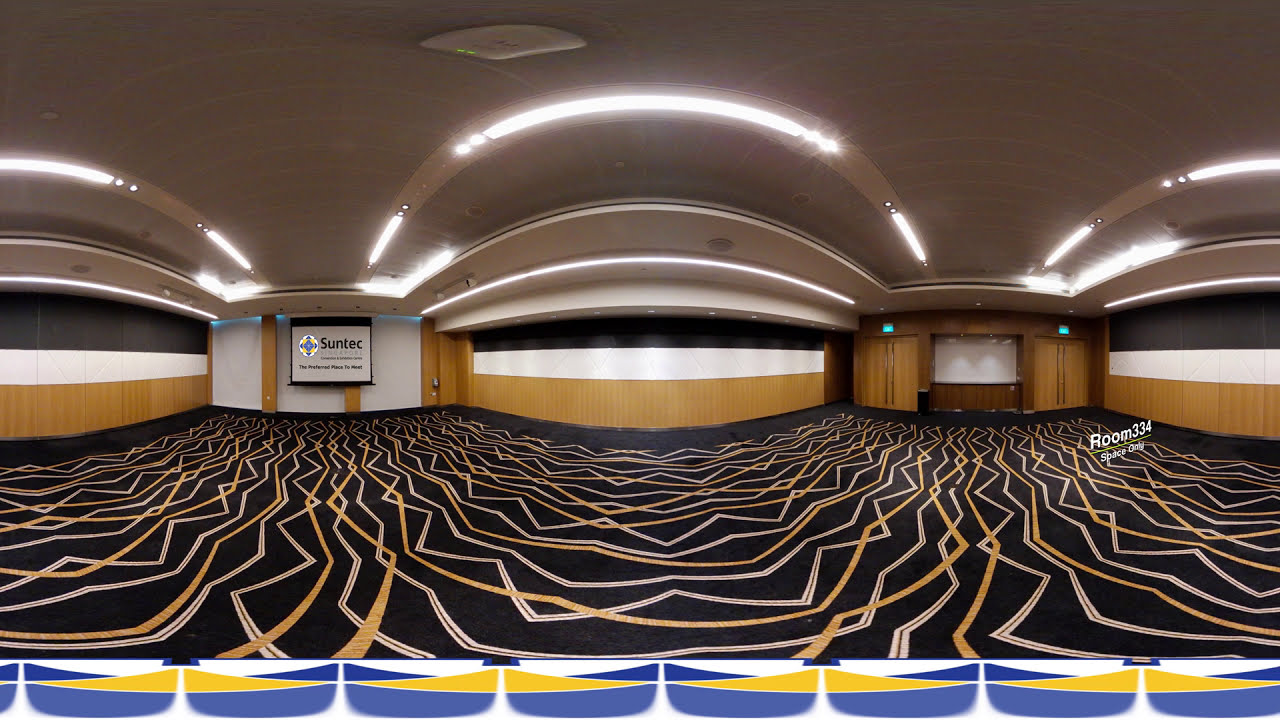The image depicts a spacious, indoor auditorium-like setting, marked by a large, carpeted floor adorned with zigzagging lines in white and yellow. These lines intersect and lead to curved areas on both sides of the room. The carpet dominates the lower half of the image, while the upper half is taken up by multicolored walls and a ceiling featuring illuminated archways. On the left side of the room, a large screen or poster on the wall displays the word "Suntech" in prominent letters, with smaller, unreadable text beneath it. To the right, another screen is flanked by brown areas that could be curtains or a stage, illuminated by two blue lights. Printed on the image, just to the right, is the text "Room 334." The overall ambiance suggests a convention or performance space, potentially captured using 360-degree technology, with some artificial editing evident in the form of yellow triangles and blue ovals at the bottom of the photo.